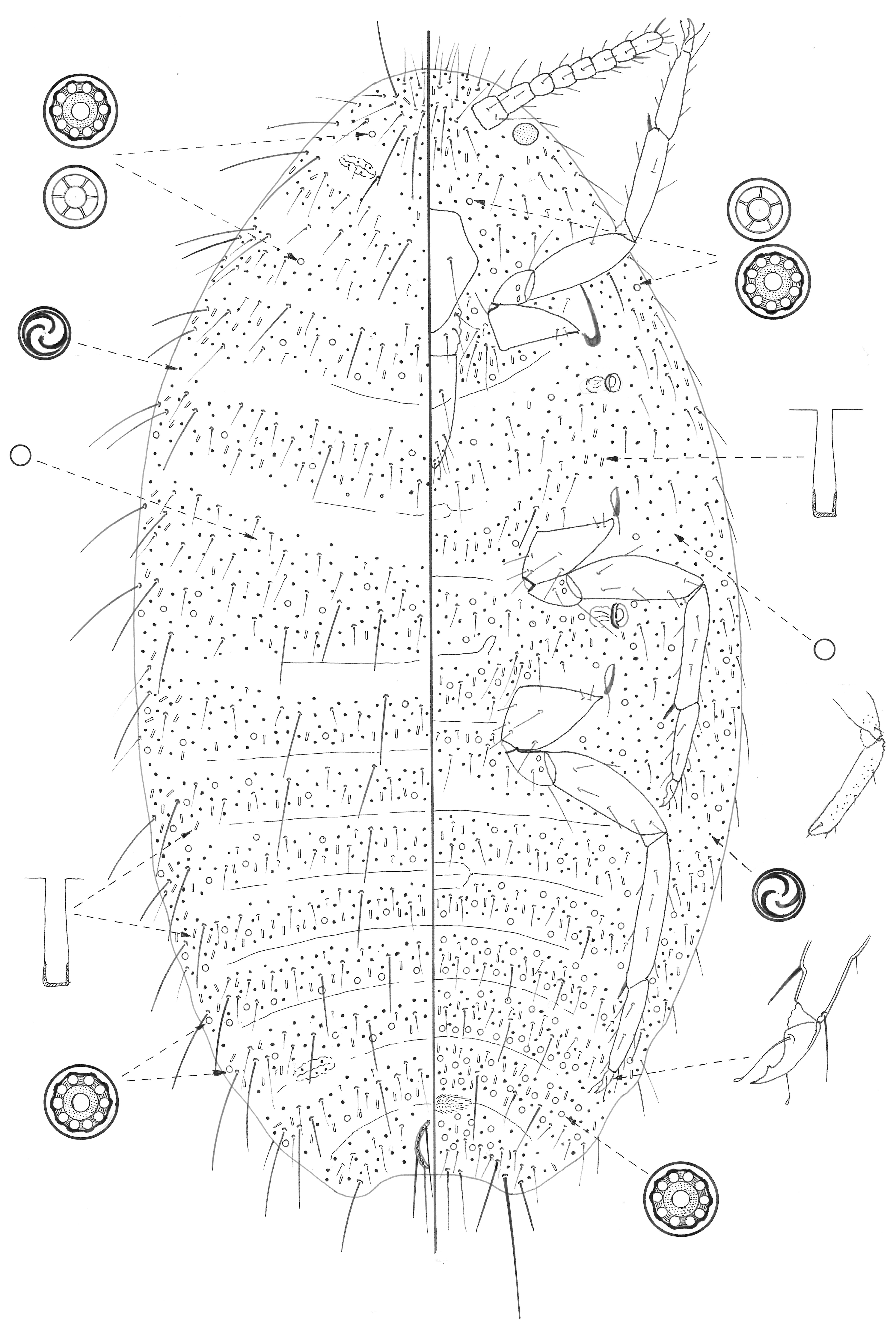The image displays a detailed, line-drawing sketch of an insect or mite against a plain white background. The entire body of the bug is formed using intricate dots and lines, possibly in shades of greens and blues. A straight vertical line splits the drawing, presenting the left side as the back of the creature and the right as the underbelly. The insect is oblong-shaped, roughly 4 inches high and 2.5 inches wide, with disconnected legs that appear in varied positions—one leg even seems to scratch its head, adding a bit of whimsical character to the otherwise scientific depiction. Along the left side, small hairs stick out, detailed with tiny dotted lines pointing to different body parts, which are circled but not labeled. The right side highlights an antenna beneath the underbelly and showcases three legs, each ending in a sort of half-claw foot, also covered in fine hairs. Despite the intricate detailing and small diagrams pointing to various anatomical features, the drawing does not specify the species or name of the creature, suggesting it to be a mite.